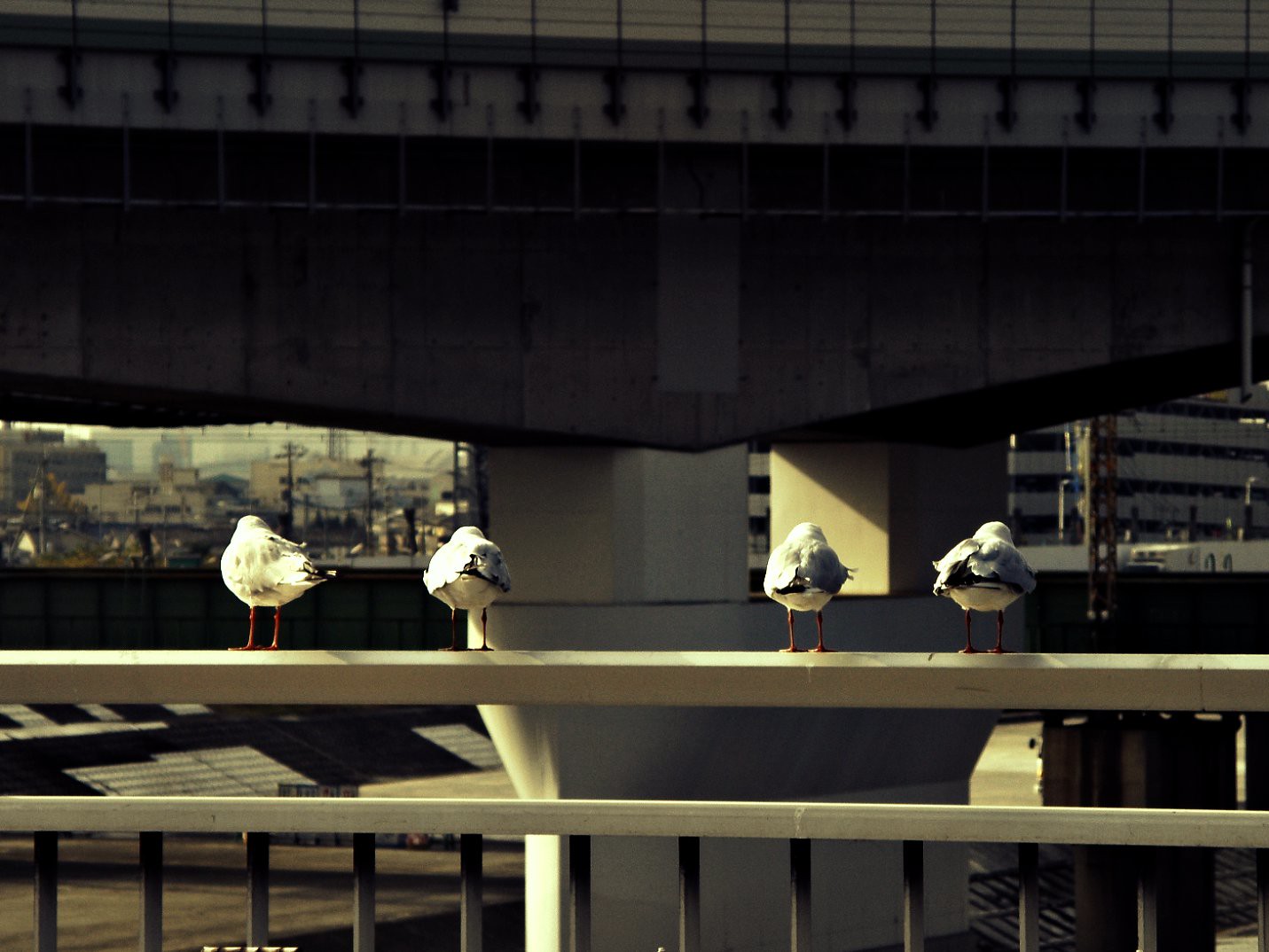This daylight outdoor image showcases a clear view of an industrial area with a cityscape in the background, comprised of varying tall and short buildings as well as some telephone poles. In the middle ground, a concrete and metal bridge or overpass spans the scene, providing a sense of depth and structure. Sitting on a stainless steel ledge in the foreground, directly beneath the overpass, are four seagulls with their backs turned to the camera. These seagulls, with white and gray plumage accented by black tail feathers, are detailed with distinctive red or orange legs. They are arranged in two pairs, each pair positioned on either side of a gap between them. The sunlight casts reflections off the steel railing and creates shadows that enhance the detail of the scene, while the overall composition suggests an urban, possibly harbor-front location.